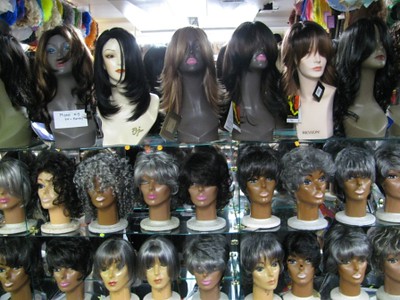This image, captured inside a wig shop, prominently features three shelves showcasing an array of mannequin heads adorned with diverse wigs. The top shelf displays longer wigs that drape to shoulder length or slightly below, featuring a mix of wavy, curly, and straight styles. The middle shelf highlights wigs with tight curls and ringlets, predominantly in shades of grey and brunette. The lower shelf is dedicated to shorter wigs, primarily in bob cuts. Each mannequin head varies in skin tone, ranging from tan to white to black, with some also bearing diverse lip shades. The arrangement places longer-necked mannequins on the top shelf, while those with shorter necks are positioned on the middle and bottom shelves. Visible price tags dangle from certain wigs, adding to the authenticity of the shop setting. The background reveals overhead lights and fabric hangings, further enriching the detailed scene.